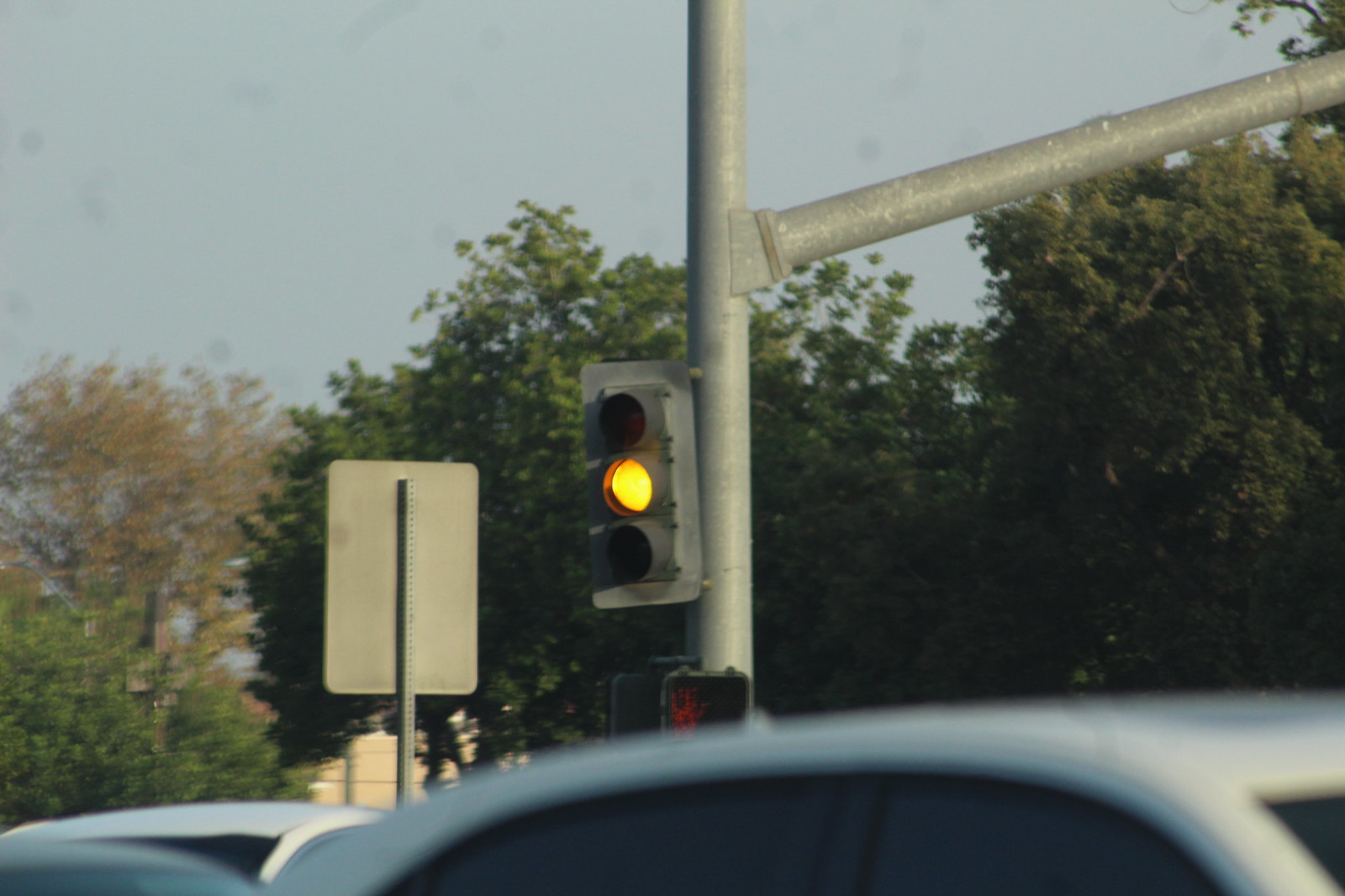The photo captures an outdoor scene featuring a traffic light and various elements of the environment. Central to the image is a black traffic light mounted on a tall silver pole; the yellow light is illuminated, while the red and green lights remain off. Directly below the traffic light, there is a crosswalk signal. Positioned to the left of the pole, an information street sign is visible, although its face is turned away from the camera, offering only the view of its gray backside. Adding to the complexity, another silver pole protrudes horizontally from the main pole, located slightly above the traffic light on its right side.

In the background, the sky appears predominantly gray with hints of blue, setting a somewhat overcast atmosphere. Lush green trees in full bloom frame the scene, their shades varying from dark to light green. The tops of several parked cars, their roofs and partly visible windows, occupy the immediate foreground. Details of a house are partially obscured by the dense foliage, and hints of the nearby road suggest mild traffic with cars potentially waiting at the light.